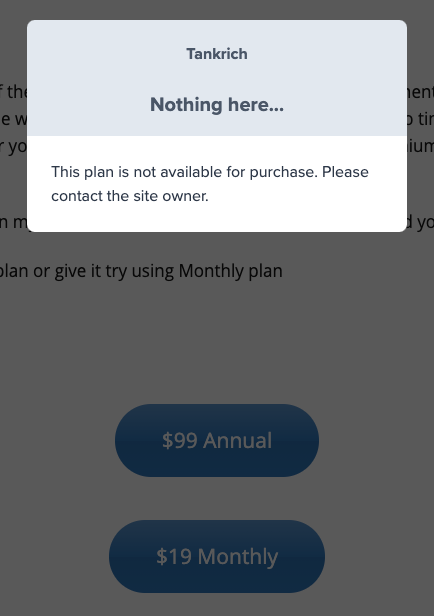This image captures a partial screenshot of a webpage featuring a pop-up window obstructing the content behind it. The pop-up message, positioned at the top of the screen, indicates a restriction and reads, "Tank rich - Nothing here. This plan is not available for purchase. Please contact the site owner." Below the pop-up, blurred but somewhat visible text suggests that the obscured page likely provides a description and sign-up options for a service plan. Underneath the pop-up window, two blue pill-shaped buttons are stacked vertically. The top button has white text that reads "$99 annual," while the button below it states "$19 monthly." Additionally, the text below these buttons reads, "or give it try using monthly plan," though partially blocked by the pop-up.